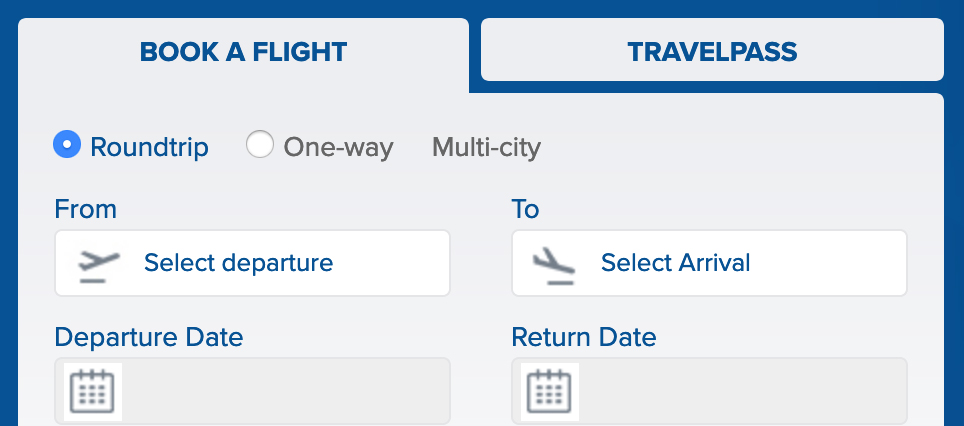The image depicts a flight booking website with a blue outline set against a white and greyish background. At the top of the interface, the word "Bokeh Flight" is prominently displayed in blue text over a grey background. Alongside it, the phrase "Travel Pass" also appears in blue text against a grey background. The highlighted option is "Bokeh Flight," indicating it has been selected. Below these options, you can choose between "Round Trip," "One Way," and "Multi-City" trips. The "Round Trip" option is currently selected, denoted by a blue circle with a white dot inside, while "One Way" and "Multi-City" are greyed out with a white circle.

The interface then prompts users to specify their flight details with "From" and "To" fields, both labels in blue text. The input boxes to select departure and arrival locations are white with blue text that reads "Select departure" and "Select arrival," respectively. Further down, fields to enter the departure and return dates are also highlighted with blue text, outlining the comprehensive process needed to book a flight.